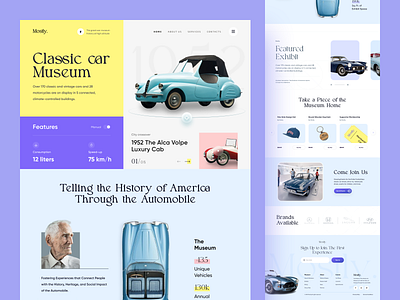The image resembles a magazine advertisement for the Classic Car Museum, encased within a 3-inch wide and 2-inch high rectangular frame. The layout features a distinct purple border that runs along the left-hand side, across the top, and down the right-hand side, creating a clear visual separation. In the upper left-hand corner, a yellow square with bold black text prominently announces "Classic Car Museum." To its immediate right is a striking, light blue, aerodynamic convertible with a black soft-top, featuring a unique scooped-in driver’s side door. Below the yellow box, a purple rectangle with white text declares "Features," while additional text nearby notes specifications such as “12 liters” and “75 kilometers per hour.” Additionally, a front-facing image of a red and white car overlays a pink background, labeled "1952, the Alco Volpe Luxury Cab."

At the bottom of the left side, black text on a blue background proclaims, "Telling the History of America Through the Automobile." This tagline underscores the museum's mission. An image of an elderly Caucasian man in a suit is also present. On the right-hand side of the advertisement, there are detailed images and information about featured exhibits, with a banner that reads "Featured Exhibit" and accompanying small text fields, though difficult to decipher. Overall, the advertisement is visually rich, featuring a blend of text, classic car imagery, and a clear call to action, ideal for attracting automotive enthusiasts.